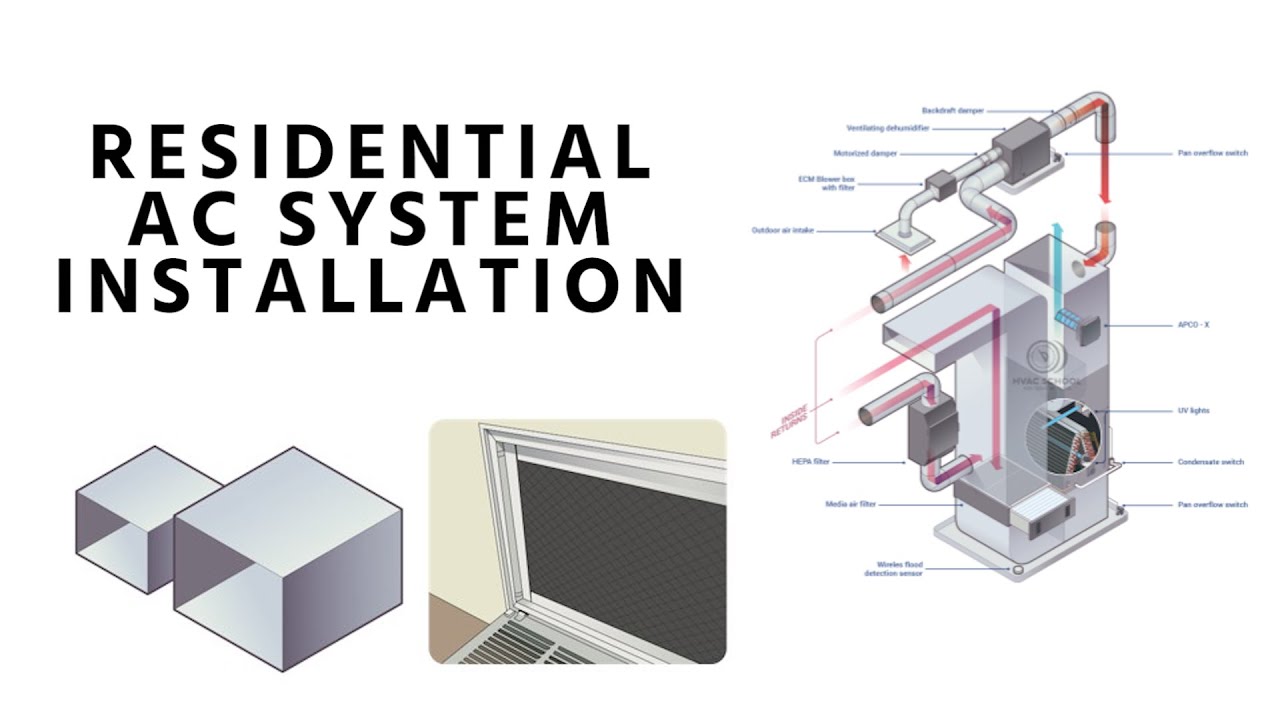The image titled "Residential AC System Installation" depicts a detailed diagram for installing an air conditioning system, with the title prominently displayed on the left side. Below the title, there are two large white cubes, which appear to be cutaway examples of air ducts. Next to these cubes is a smaller image of an open vent, seemingly unfastened at the top and opened outward while still attached at the bottom. The right side of the image features an intricate, exploded view of an HVAC unit. This technical cutaway diagram reveals every individual part of the unit, all meticulously labeled, showcasing the connections between components. The diagram includes arrows to illustrate airflow direction, with red arrows indicating hot air and blue arrows denoting cool air. The entire scene is set against a white background with black text, resembling a detailed instructional guide that you might find in a textbook.